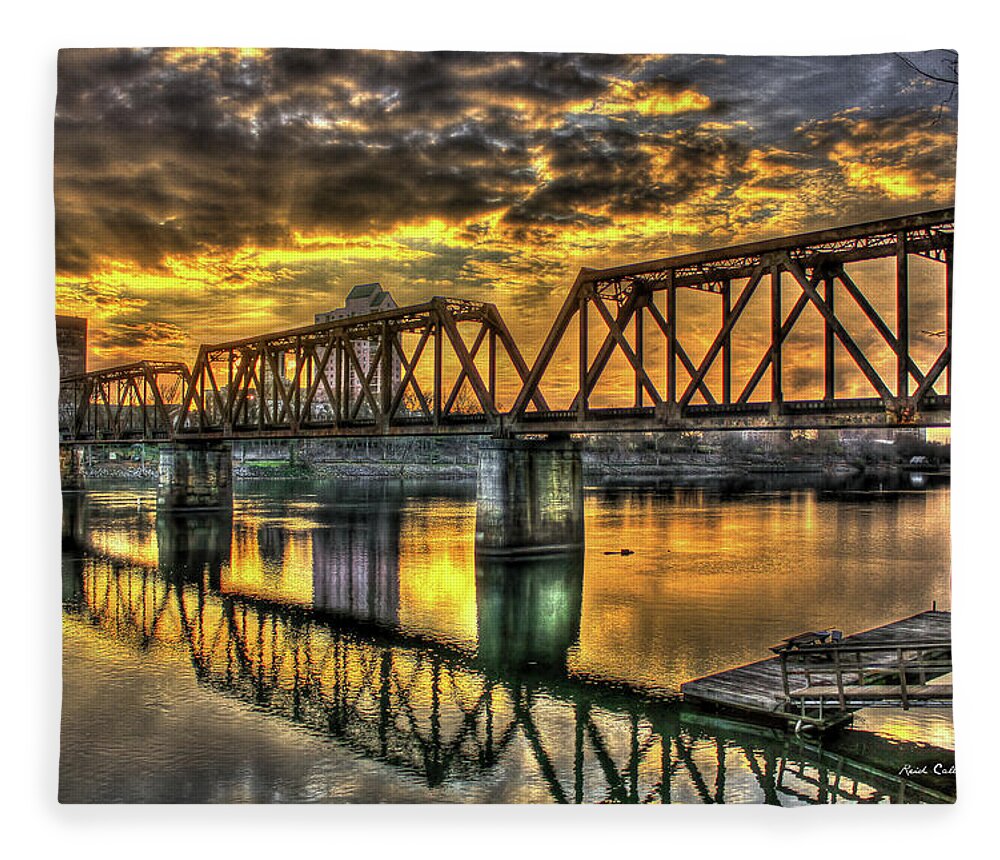In this photographic image, the scene is set outdoors during an enchanting sunset. A meticulously crafted iron bridge, featuring three trapezoidal sections and intricate metal work, stretches across a calm body of water in a city. The bridge is supported by solid concrete pilings that extend from the water's floor. The surface of the water below, tinted red and brown by the setting sun, mirrors both the bridge and the dramatic skyline above. 

The sunset sky is a spectacle of its own, adorned with vast, thick, black clouds with golden edges, casting beams of light and flecks of gold through breaks in the cloud cover. This illumination causes the water to appear almost like a serene lake. In the background, a multi-story brown building with two prominent gable roofs stands tall, alongside a structure that may be utilized for grain storage. At the bottom right corner of the image, a dock and gangway are visible, hinting at a point for boats to be boarded.

The overall ambiance, with the absence of any textual distractions, conveys a beautiful yet foreboding atmosphere, as the clear reflections in the still water add to the photograph's remarkable and tranquil detail.